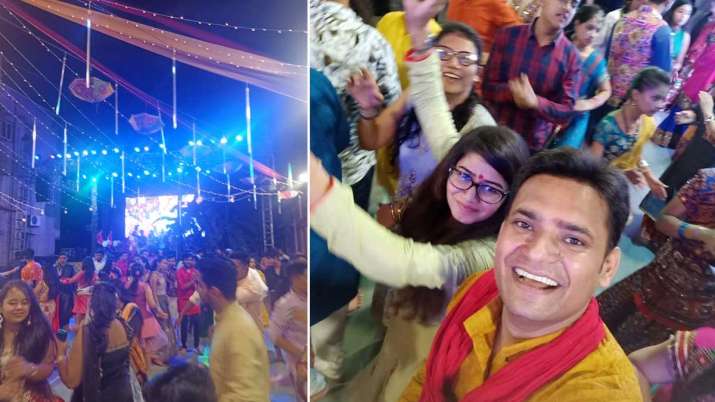This is a two-paneled image capturing a lively Indian wedding celebration. The photograph on the left shows a vibrant scene with numerous people dancing under a canopy of colorful decorations including umbrellas, ribbons, and beads hanging from the ceiling. The atmosphere is illuminated by an array of blue, orange, and purple lights that add to the festive ambiance. A large stage adorned with digital artwork is visible in the background. Most attendees are dressed in traditional Indian attire, featuring bright yellow, red, and mustard colors, enhancing the grandeur of the event. 

The right panel displays a close-up of a man taking a selfie with a woman, both smiling joyfully. The woman, who has long brown hair, is wearing black glasses and a bindi (red dot) on her forehead. Both are clad in traditional clothing, with the man in a checkered red and black shirt and the woman in bright, festive colors. Surrounding them are more guests attired in similarly vibrant outfits, contributing to the overall joyous atmosphere of the celebration.